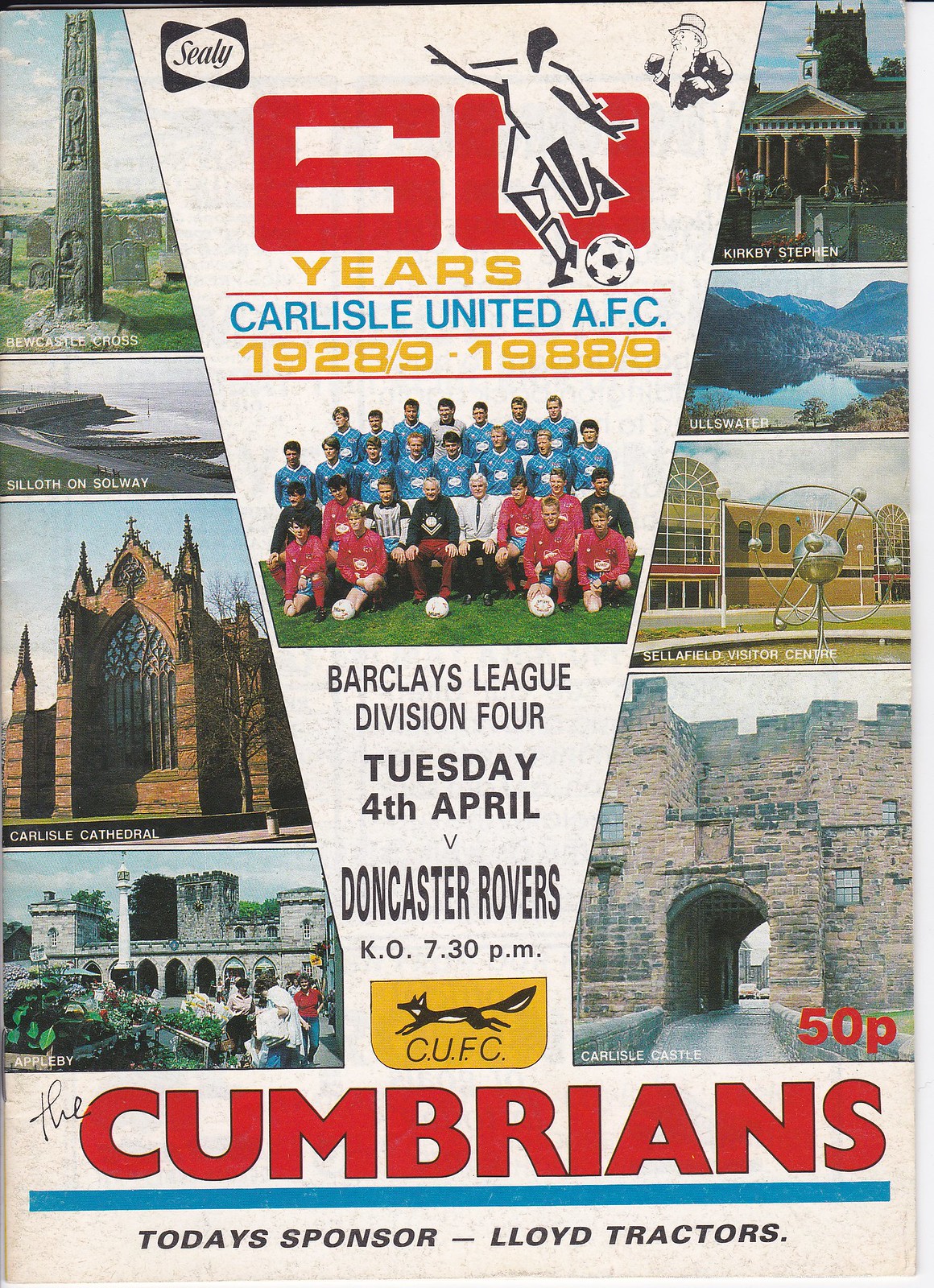The magazine cover for a sports event prominently features a solid white background with "The Cumbrians" in big red letters at the bottom, above a solid blue line. Below this line, in black text, it reads "Today's sponsor: Lloyd Tractors." Central to the layout is the Sealy symbol, commemorating "60 years of Carlisle United AFC 1928/9 – 1988/9." The cover also includes a photograph of a football team in their jerseys with the text "Barclays League Division 4, Tuesday 4th April vs. Doncaster Rovers, KO 7:30 p.m." Additionally, the cover is adorned with multiple images of landmarks: the top left features Bewcastle Cross with a large pillar carved with human figures, a rocky grey beach labeled "Siloth on Solway" below that, and the front of Carlisle Cathedral. The images, numbering about eight, include various buildings, waterlines, and archways, set against a palette of white, black, red, brown, gray, blue, yellow, and green. This detailed, vibrant cover serves as a program for a football game, blending historical landmarks with sports commemorations.